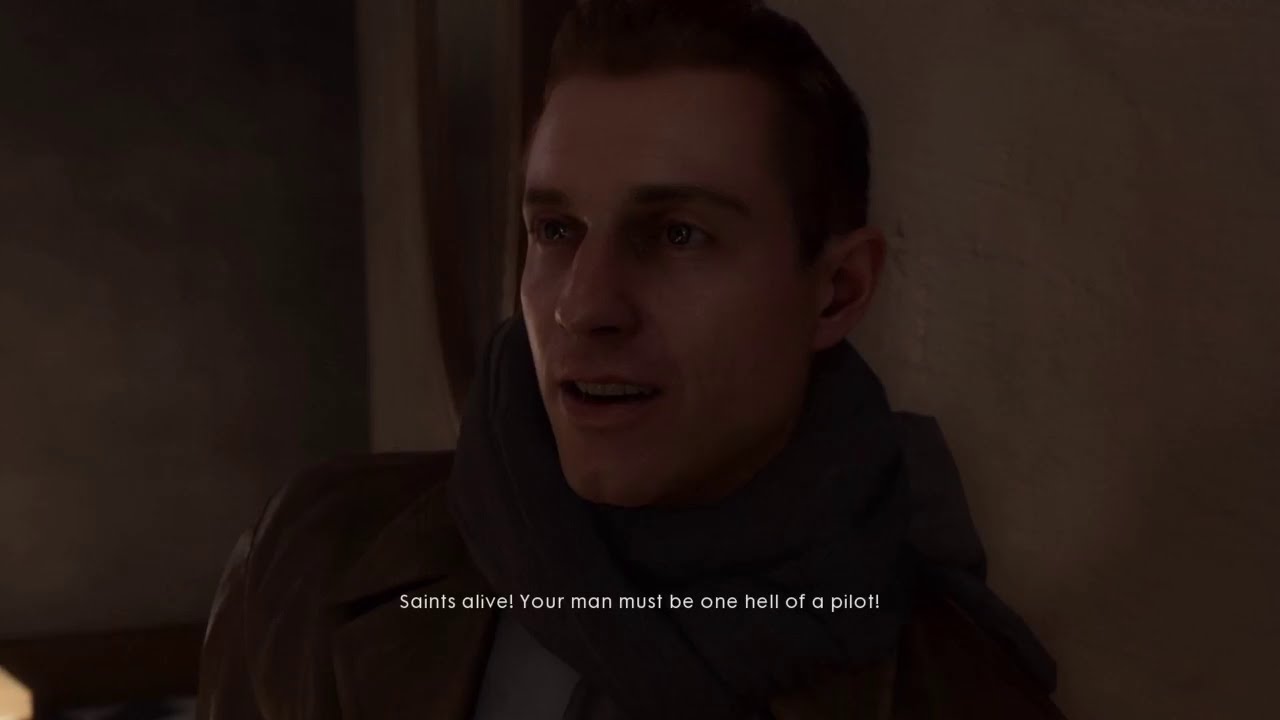This detailed photograph, seemingly a still from a video game, portrays a well-dressed Caucasian gentleman in his 30s, centered in the image with his head and shoulders visible. The color palette is dominated by various shades of brown, casting a warm, almost sepia tone over the scene. The gentleman has short brown hair, brown eyebrows, and possibly blue eyes, though brown is also suggested. His features include a straight, thin nose, a slight dimple on his chin, and lips described as thin on the upper and fuller on the lower, with his mouth slightly open, revealing the top row of his teeth, as if caught mid-sentence or in contemplation. He dons a brown jacket with prominent collars over a gray scarf wrapped snugly around his neck, further enhancing the warmth of his outfit. The backdrop consists of brown walls that appear to be plaster or sandstone, positioning him in what seems to be a corner of a room. Below his serene yet pondering face is the white, small-text caption: "Saints alive, your man must be one hell of a pilot!" adding context and character to the composition.